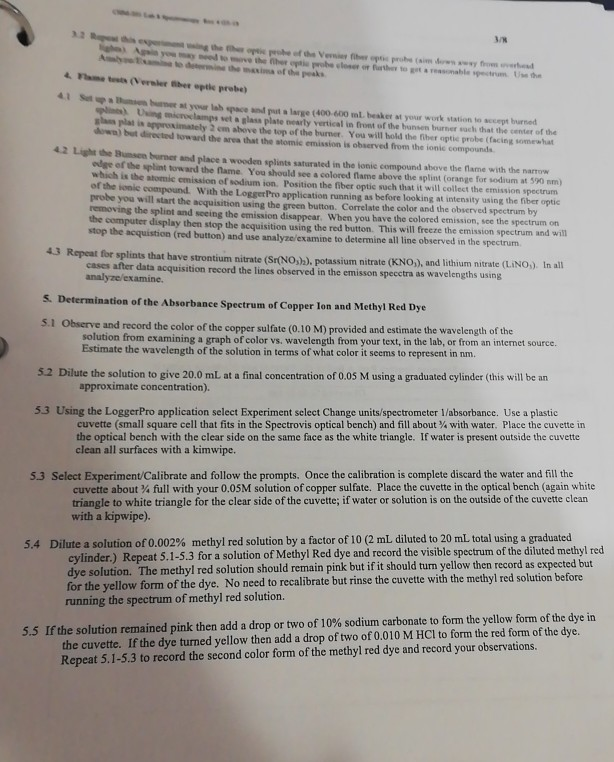The image captures a close-up view of a page from a scientific document, likely related to a chemistry class or experiment, securely held in a binder. The binder's metal ring is visible in the top right corner, and the page is riddled with hole punches. Though the text on the paper is mostly out of focus, it includes identifiable sections and instructions. The page is marked as page 3 out of 8 in the top left corner, indicating it is part of a larger document. The visible sections include parts of various instructions and headings referring to a "flame test" and "Vernier fiber optic probe," as well as detailed steps under section 5 titled "Determine the absorbance spectrum of copper ion and methyl red dye," with bullet points ranging from 5.1 to 5.5. There is a specific instruction about observing and recording the color of copper sulfate, estimating the wavelength based on a color versus wavelength graph, and preparing a diluted solution to a specified concentration. The document appears to be a part of a chemistry lab report or manual, featuring detailed experimental procedures written on white paper with black text.